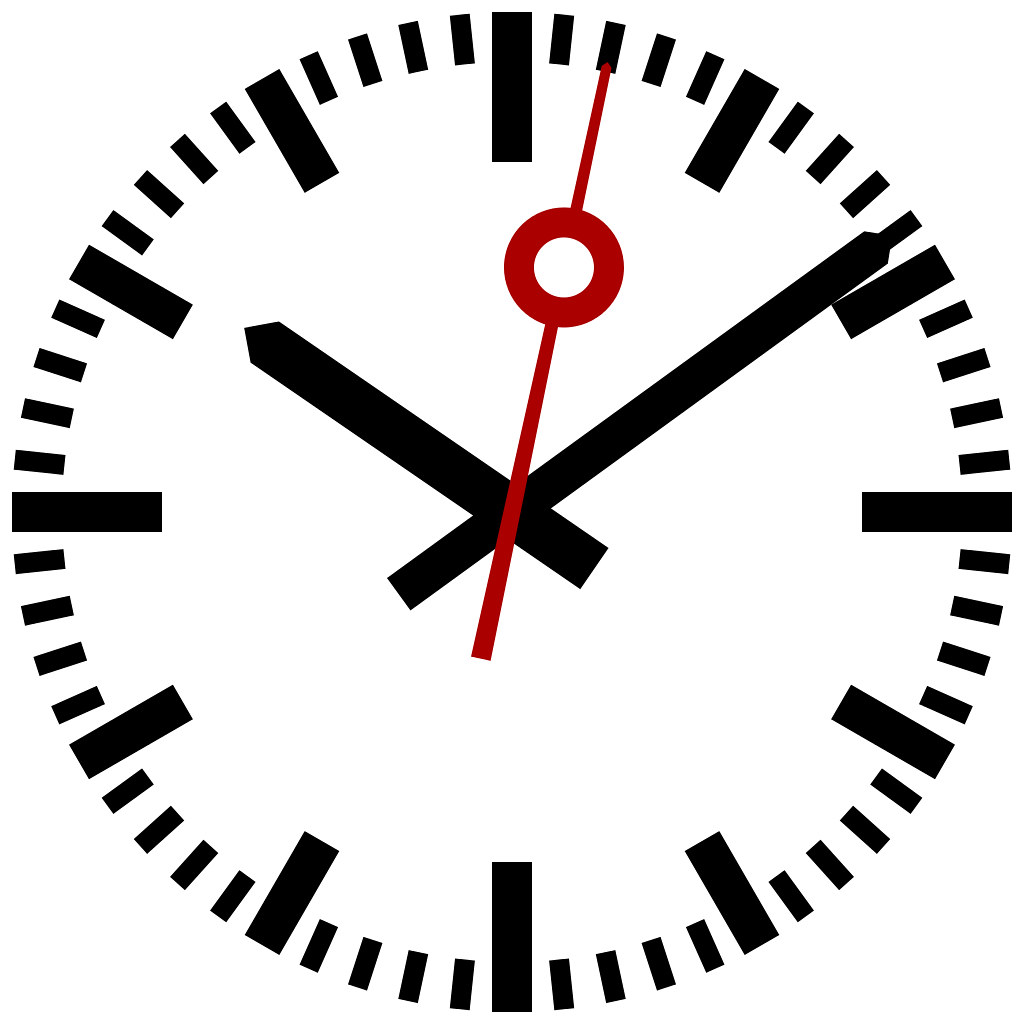This image resembles clip art of a clock face, characterized by its minimalist design devoid of any numbers. Instead, thick black rectangles mark the positions where the numbers would traditionally be, with smaller black rectangles in between these larger markers. The central axis features two primary hands: a shorter, rectangular hand with a pointed arrow edge indicating the 10 o'clock position, and a longer hand pointing just before the 2 o'clock mark. Additionally, a distinctive red hand, complete with a circular element in its middle, is also present on the clock face.